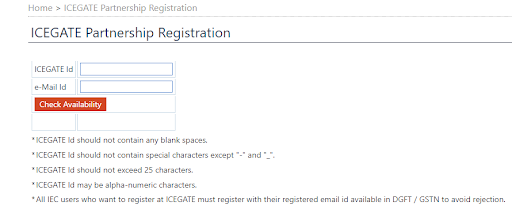The image depicts a registration panel for the IceGate partnership. At the top of the panel, there is a navigation trail starting with "HOME," followed by an arrow leading to "ICEGATE" in all caps, and ending with "Partnership Reg." Below a thin gray line, "Partnership Registration" is prominently displayed in larger black text. Just beneath this heading is a darker gray line.

Lower on the panel, the text "ICEGATE ID" is visible next to an input field with a thin blue border. An "Email ID" input field is also present. Beneath these fields is a red button labeled "Check Availability." 

Further down, the panel includes several blank fields followed by a series of registration guidelines, each beginning with an asterisk:
- ICEGATE ID should not contain any blank spaces.
- ICEGATE ID should not include any special characters except dashes and underscores.
- ICEGATE ID should not exceed 25 characters.
- ICEGATE ID may consist of alphanumeric characters.
- All IEC users must register with the email ID already registered in DGFT/GSTN to avoid rejection.

The background of the panel is plain white with no additional branding or graphics.